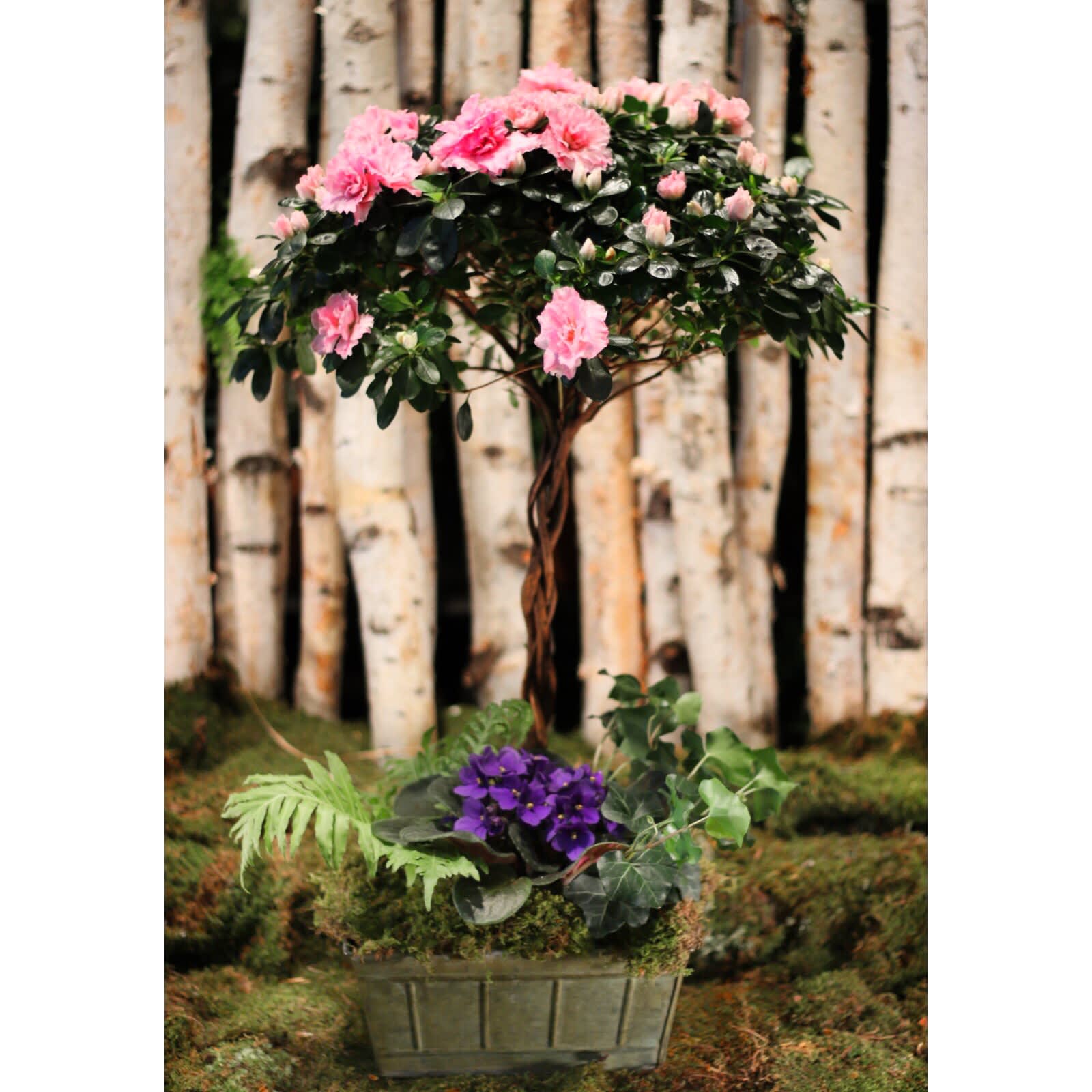This image showcases a small, flowering tree seated in a square planter with a greenish-brown hue. The lush base of the planter is adorned with ivy, ferns, and a striking African violet. Rising from the verdant base, the trunk ascends and blossoms into a crown of waxy, dark green leaves interspersed with vibrant, multi-petaled pink flowers, resembling a camellia bush. The arrangement is positioned on a mossy surface, lending a natural and serene atmosphere. In the backdrop, there are tall, slender tree trunks clad in white bark with patches of black and orange, contributing to the ethereal ambiance of the scene.